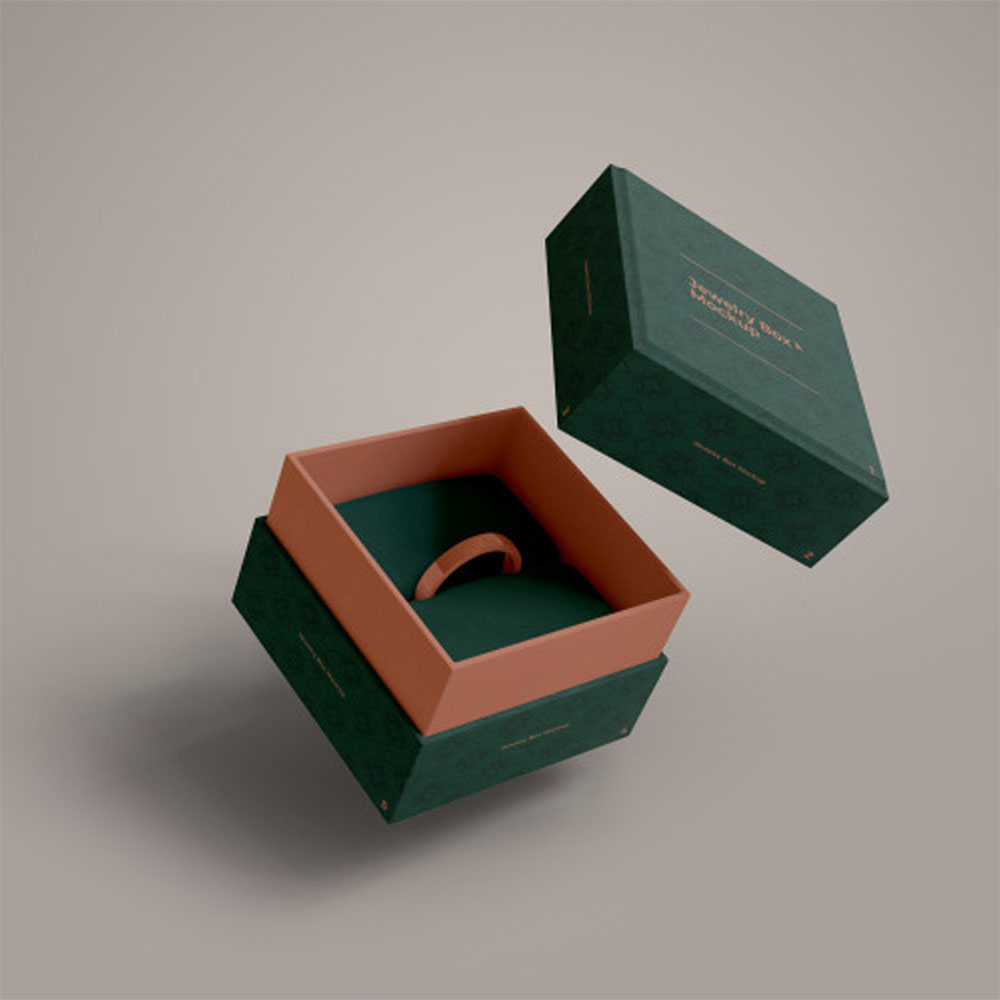This is a detailed photograph of a green, marble-textured jewelry box set against a featureless gray background. The box appears to be slightly elevated above the surface, casting a shadow below. The lid of the box is floating above it at an irregular angle. The exterior of the box is forest green with two gold lines on the top, and between these lines, in gold font, it reads "Jewelry Boxes Mock-up" with additional smaller writing on the side. The interior sleeve, where the top of the box fits over the rest, is a tan salmon color. Inside, the box has a green bed with a crease where a golden ring, made from a plastic-like polymer, is embedded, with just the top half visible and facing upwards. The overall presentation is elegant and refined, highlighting both the box and its contents.